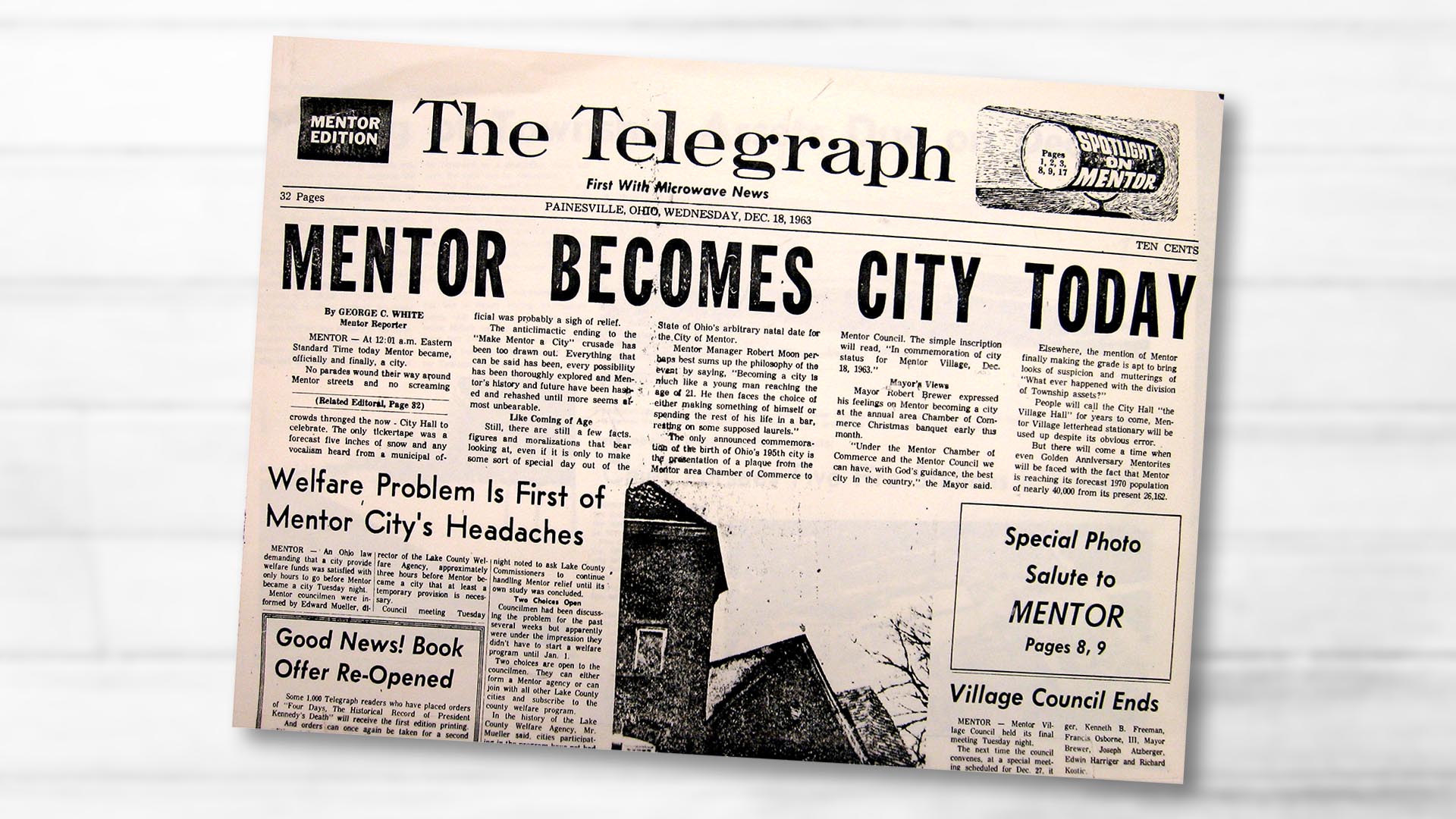The front page of a vintage newspaper titled "The Telegraph: Mentor Edition," printed on Wednesday, December 18, 1963, in Painesville, Ohio, proudly announces Mentor's transition from a village to a city. At 12:01 a.m. Eastern Standard Time, Mentor officially became Ohio's 195th city, markedly without parades or throngs of celebratory crowds—only the forecasted five inches of snow and a collective sigh of relief from municipal officials marked the occasion. George C. White, Mentor Reporter, details this historic moment in his article, "Mentor Becomes City Today." Mayor Robert Brewer and Mentor Manager Robert Moon reflect on the significance of city status, anticipating its growth from a population of 26,162 towards a forecasted 40,000 by 1970. A plaque was presented by the Mentor Area Chamber of Commerce to commemorate the milestone. The newspaper, spanning 32 pages and costing 10 cents, highlights other local news including the headline "Welfare Problem is First of Mentor City's Headaches," elaborating on the council's recent decision to seek temporary welfare management from Lake County. Additionally, "Good News Book Offer Reopened" informs readers about the availability of a historical record on President Kennedy's death. Prominently featured on pages 8 and 9 is a "Special Photo Salute to Mentor," celebrating this significant event in Mentor's history.